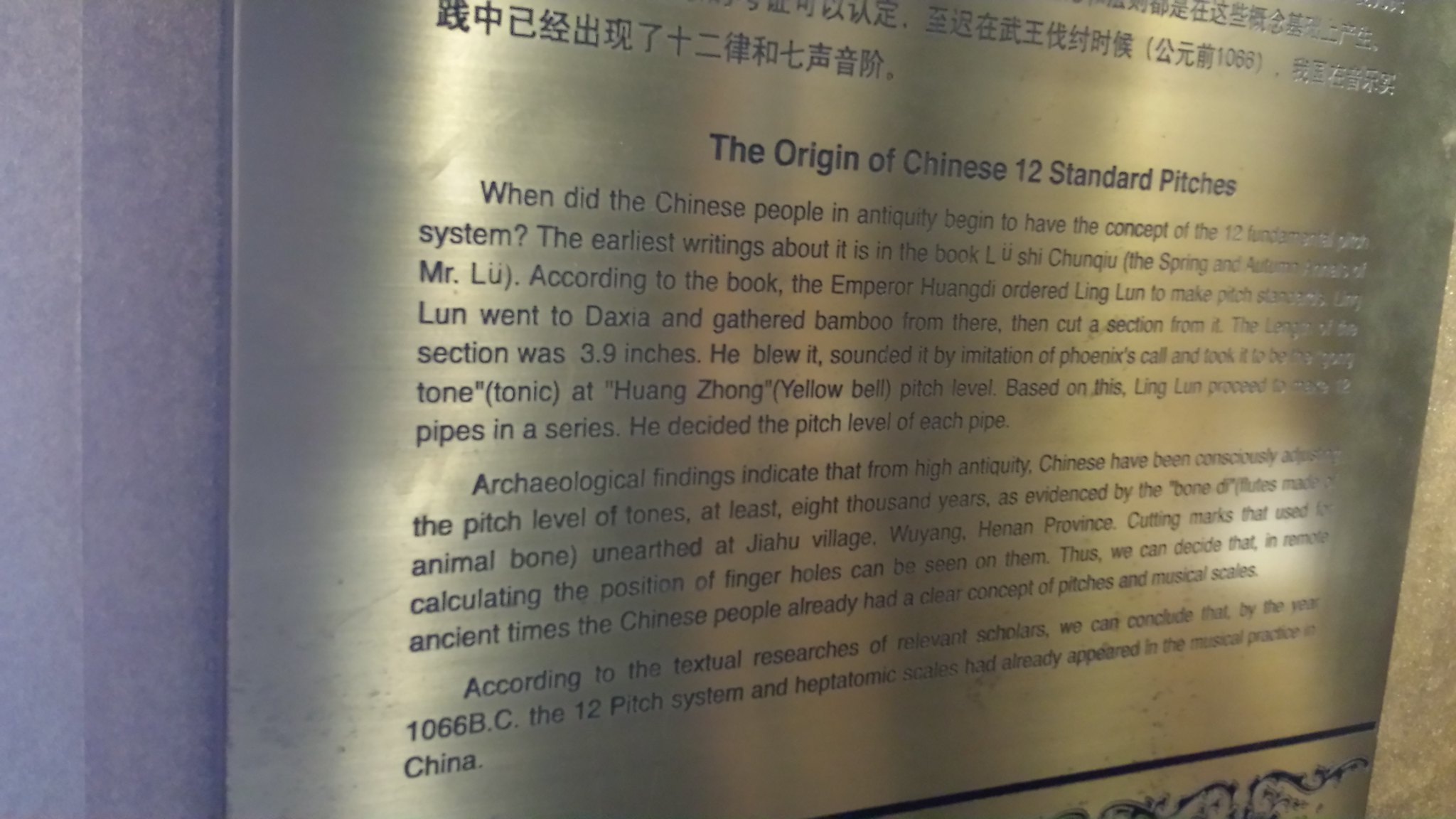This image displays a light golden plaque prominently featured against a white concrete wall in a museum setting. The plaque, which occupies most of the space in the image, is primarily written in black with Chinese characters at the top. Below this, a bold, black subheading in English reads, "The Origin of Chinese Twelve Standard Pitches." The explanatory text, divided into three paragraphs, delves into the historical concept of the twelve-pitch system in ancient China. Although the full text is partially obscured due to glare and blurriness, it starts with, "When did the Chinese people in antiquity begin to have the concept of the twelve-fundamental pitch system?" It continues to reference historical documents such as the "Book of Lu Shi" and "Penghai, The Spring." This plaque serves to inform visitors about the archaeological findings related to the origins and development of the twelve-pitch system in Chinese culture.